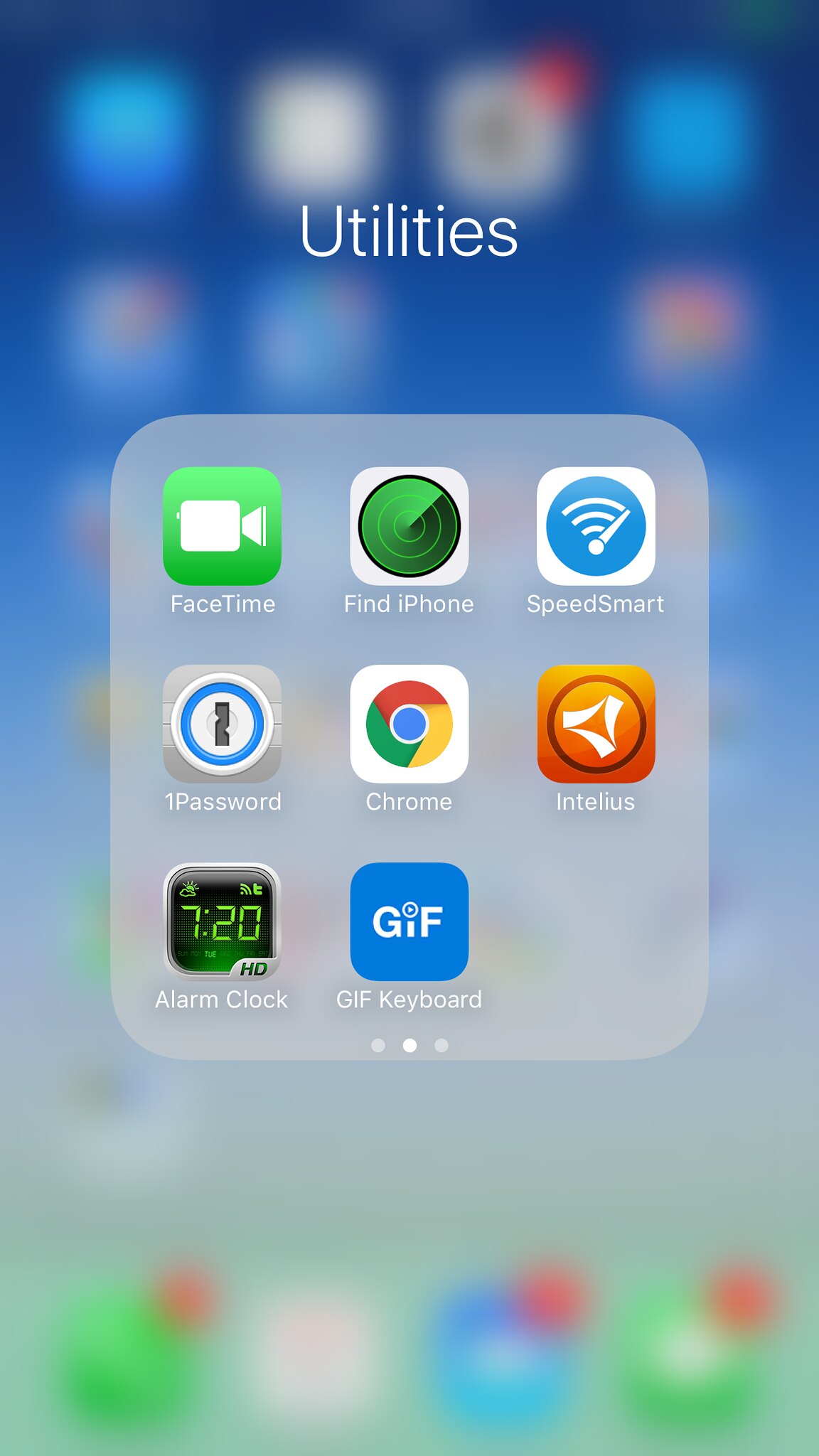The screenshot captures a smartphone display featuring an open 'Utilities' folder against a predominantly blue background with blurred icons. Dominating the top of the screen, the word 'Utilities' appears in a thin sans-serif font. Below, the rounded-corner folder box contains an assortment of apps:

- The top row starts with a green box featuring a camera icon labeled 'FaceTime.'
- Next, a white box with a green circle resembling a radar, labeled 'Find iPhone.'
- Adjacent to it, a white box displaying a Wi-Fi symbol and an arrow pointing right with 'SpeedSmart' beneath it.

In the second row, from left to right:
- An icon that resembles a lock and key, labeled '1Password.'
- In the middle, the icon for the Chrome browser, labeled 'Chrome.'
- To the right, an orange-red icon with triangular shapes and a white circle in the center, labeled 'Intelius.'
- A green icon with a clock showing 7:20 and a corner marked 'HD,' labeled 'Alarm Clock.'
- The last icon features a blue box with the letters 'GIF' and is labeled 'GIF Keyboard.'

At the bottom of the folder box, three navigation dots are displayed, with the middle dot highlighted in white, indicating the current screen, while the side dots are faded.